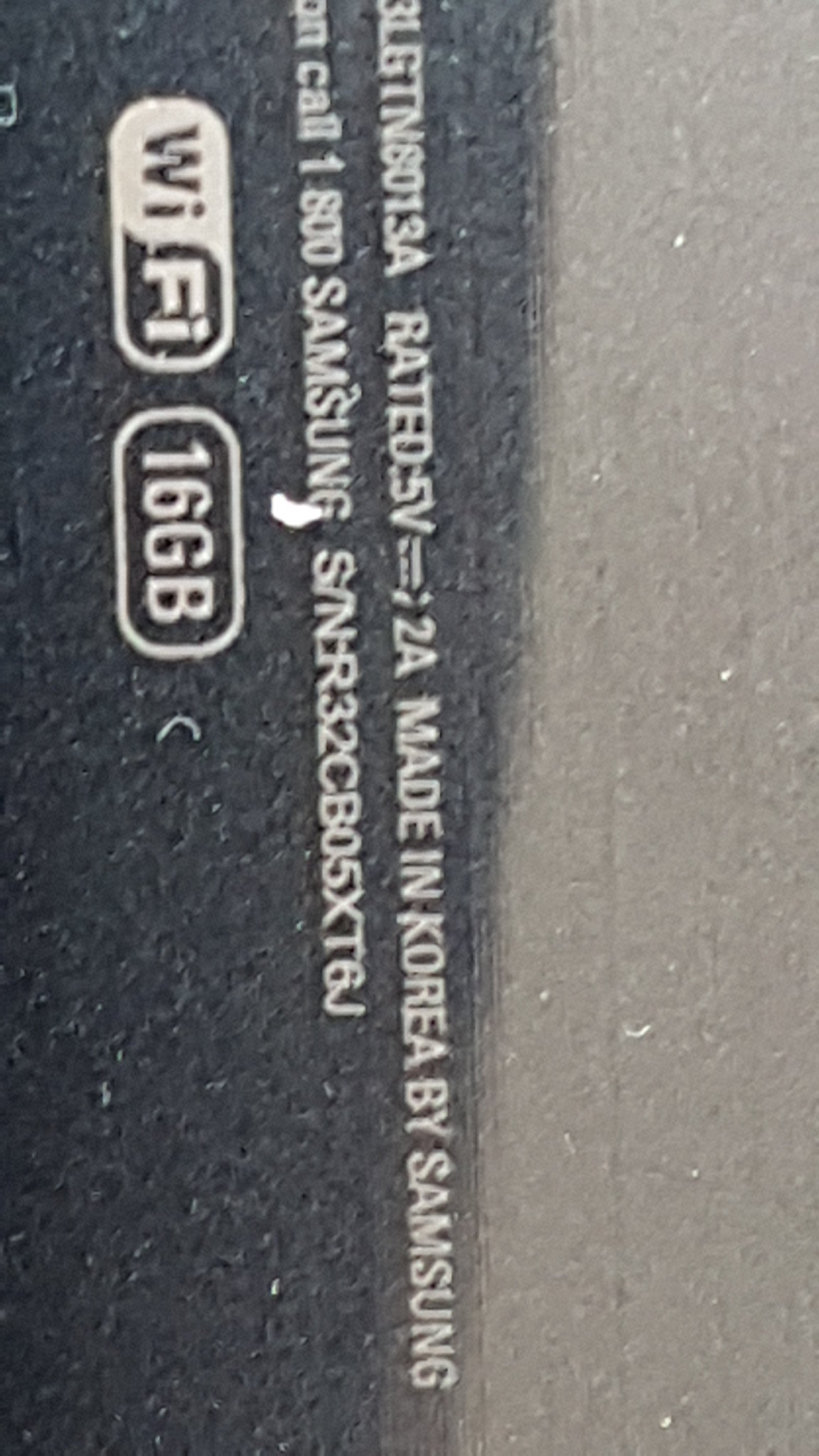The close-up color photo features a section of electronic equipment with various text details. The image has been vertically rotated, requiring a 90-degree counterclockwise rotation for proper horizontal alignment. The photo, taken in a sunny room, displays a stark contrast between the sunlit and darker portions, with a gray and black background. The equipment bears partially chopped-off labeling, including "LGTN 8013A," "rated 5V 2A," and "made in Korea by Samsung." The writing is white, though some areas appear washed out due to sunlight. Additional text includes a contact number "1-800-SAMSUNG" and a serial number "S/N 32CB05XT6J." Also present are two distinctive symbols: a yin-yang styled Wi-Fi icon, and an oval outline with "16GB" inscribed within it. The image is somewhat grainy and contains small white particles, possibly dust.